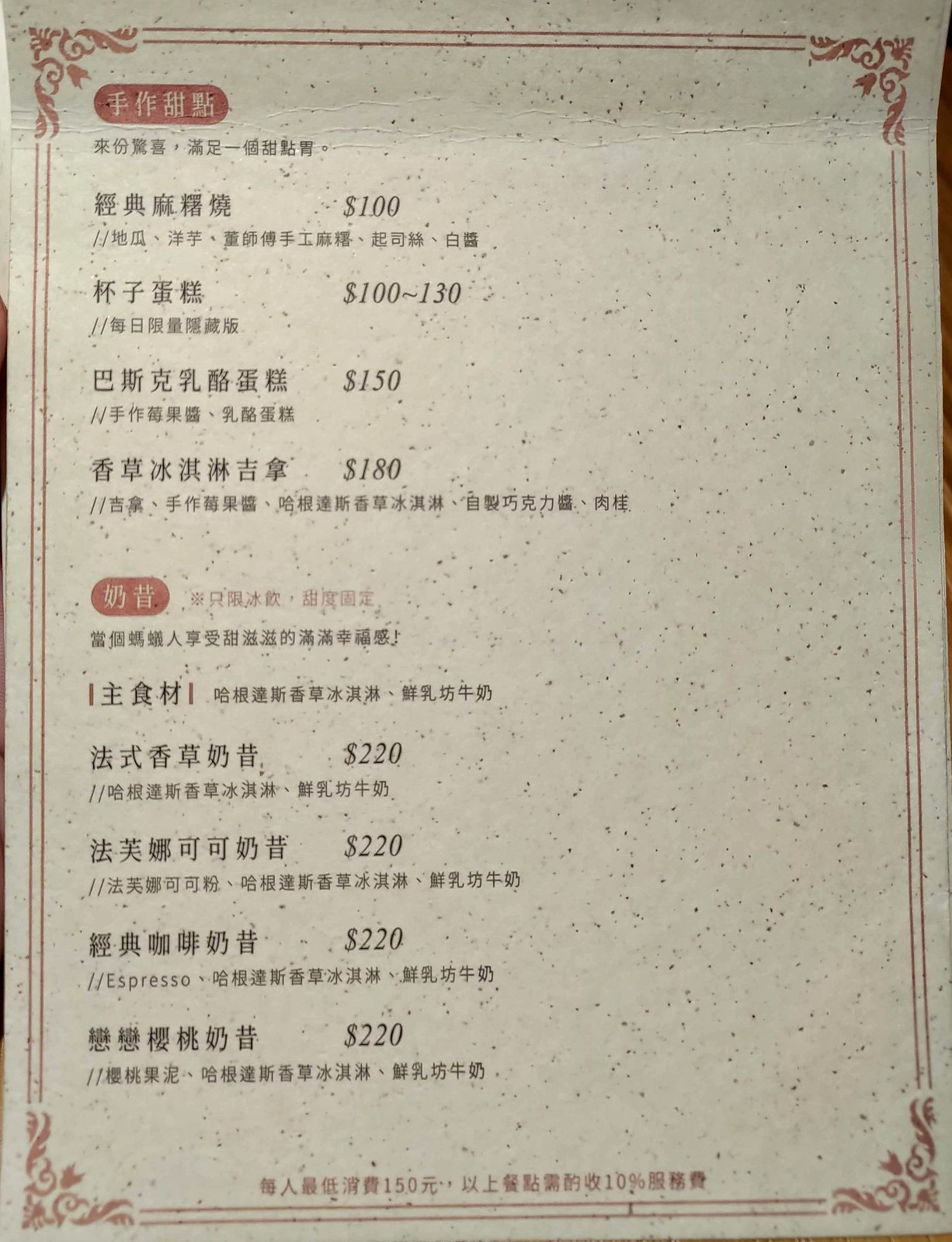This photograph features a rectangular piece of gray paper adorned with numerous black speckles, resembling the texture of a traditional menu. The menu is framed within a double-line rectangular border, which adds a refined touch to its design. Intricate curly-Q elements embellish each corner, enhancing its aesthetic appeal.

The content of the menu is written in black font, showcasing Asian characters arranged from left to right, deviating from the traditional top-to-bottom orientation. Each line of text is accompanied by a corresponding price, denoted with a dollar sign ($). At the top, the first price is listed as $100, followed by subsequent prices of $100-$130, $150, and $180. As the menu progresses, multiple lines of Asian writing continue, culminating in consistent prices of $220 listed across several lines. This intricately designed menu likely presents a variety of items, each represented through thoughtful typography and meticulous layout.